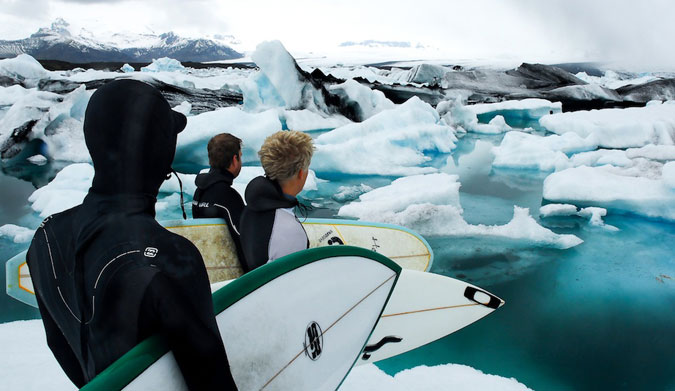In this striking color photograph, three male surfers, clad in black wetsuits, stand on a snowy iceberg amidst a frigid, dark blue ocean dotted with icebergs. Positioned in the bottom left corner, the group is enveloped by a vast, frozen landscape under an overcast sky. One surfer, foregrounded, grips a white surfboard with a green rim, his hood pulled over his head. The other two, with hoods down, reveal one to be blonde and the other brunette. The blonde surfer holds a white pointed surfboard, while the brunette clutches a round-nosed yellow board edged with blue. The expansive backdrop features a large, snow-covered mountain in the top left corner and ice floes scattered across the turquoise-tinted water, accentuating the surreal collision of surfing culture with an arctic environment. The image evokes a sense of chilly adventure, blending reality with elements that suggest photo-manipulation.